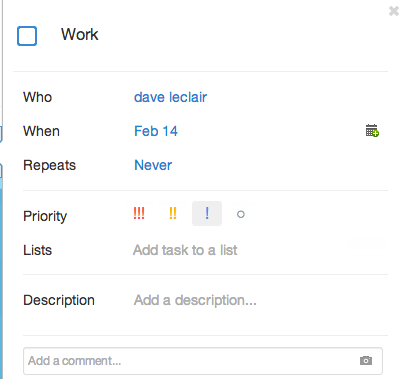This is a detailed screenshot of a smartphone reminder app. At the top left corner, it features a blue square with a white center. To the right of this icon is the word "Work," indicative of the category or list to which this reminder belongs. On the far right side of this header is a closeout "X" icon for closing the task view.

Directly below this header is a thin, light gray line, separating it from the main content. Following this separator, there are the fields labeled "Who," "When," and "Repeats." To the right of "Who" is the name "Dave LeClaire," indicating the assignee or creator of the reminder. Beside "When," the detail "February 14th" is noted with a small calendar icon next to it, marking the due date of the task. To the right of "Repeats," it specifies "Never," meaning this task does not recur.

Another light gray line further segments the content. Below this, the fields "Priority" and "Lists" are displayed. To the right of "Priority," three icons indicate urgency: three red exclamation points (highest priority), two yellow exclamation points (moderate priority), and one blue exclamation point (low priority). Correspondingly, to the right of "Lists" is the option "Add task to a list," suggesting the flexibility to categorize the task further.

A subsequent light gray line introduces the "Description" field. To the right of "Description," it prompts the user to "Add description," inviting additional task details. Below this, a comments box is available, likely for notes or additional context, accompanied by a camera icon on the right, suggesting the option to attach images.

The overall layout is clean and well-organized, providing a clear structure for managing tasks and reminders.